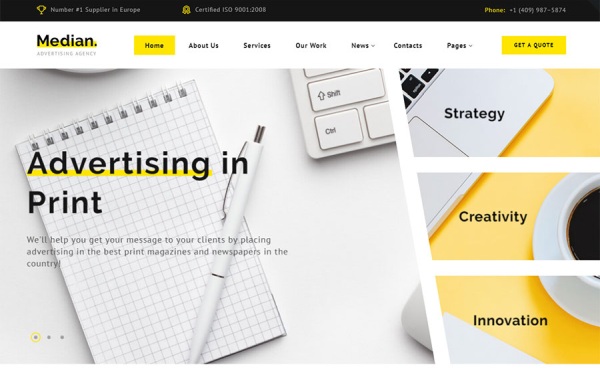On the advertising agency website, the primary color scheme features a predominantly white background accented with black text and touches of gold, reminiscent of a mustard yellow hue. At the very top of the page, various submenus are arranged from left to right across the banner. Positioned in the upper left corner, the company logo, "Median," appears in bold black block print, distinguished by a yellow highlighter effect beneath it. Beneath the logo, the phrase "advertising agency" is displayed in subtle gray print.

Across the top of the screen, the submenus include: "Home" (highlighted in mustard yellow as the current selection), "About Us," "Services," "Our Work," "News," "Contacts," "Pages," and a conspicuous yellow "Get a Quote" button. 

Dominating the main content area, just below the header, is the large black text "Advertising in Print" with the same yellow highlighter effect beneath it. This title overlays an image featuring a coil-bound graph paper notebook with a white pen resting atop it, and the corner of a calculator peeking into the frame, all set against a predominantly white background. Beneath this title, the text reads, "We'll help you get your message to your clients by placing advertising in the best print magazines and newspapers in the country."

On the right side of the page, occupying about a third of the width, there is a section split by a diagonal line featuring three vertical blocks labeled "Strategy," "Creativity," and "Innovation" from top to bottom, each set against a yellow background. This section also includes visuals of a white coffee cup and the edge of a laptop computer.

The detailed and thoughtfully designed layout underscores the agency's commitment to clear communication, strategic planning, and innovative solutions for print advertising.